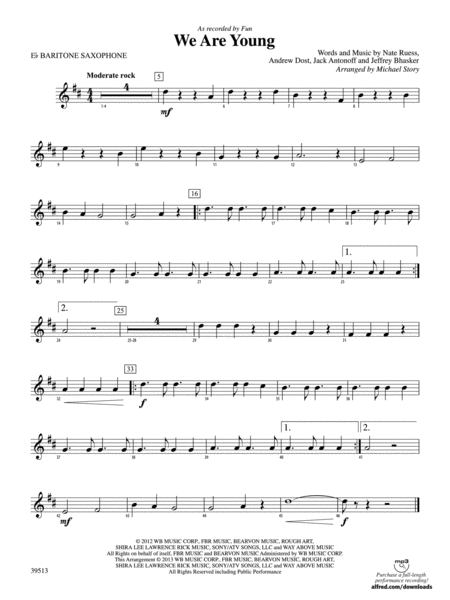This image depicts a single page of sheet music for the song "We Are Young" by the band Fun., arranged for E-flat baritone saxophone. The top of the page notes it is "as recorded by Fun," and specifies the instrument and genre: E-flat Baritone Saxophone in Moderate Rock. The musical notation is written in the treble clef with two sharps on the clef. The composer credits on the top right corner list the creators of the song: Nate Ruess, Andrew Dost, Jack Antonoff, and Jeffrey Bhasker, with an arrangement by Michael Story. The page contains eight rows of musical notation depicted on a white background in black ink. Additional text at the bottom includes copyrights from 2012 WB Music Corporation, FRR Music, Bergen Music, Buch Art, and a note about an MP3 for purchase: "Full Length Performance Recording Available at alfred.com/downloads." There's a logo on the bottom right with some words underneath it, and about six rows of black text at the very bottom of the music notation, which are partially readable.